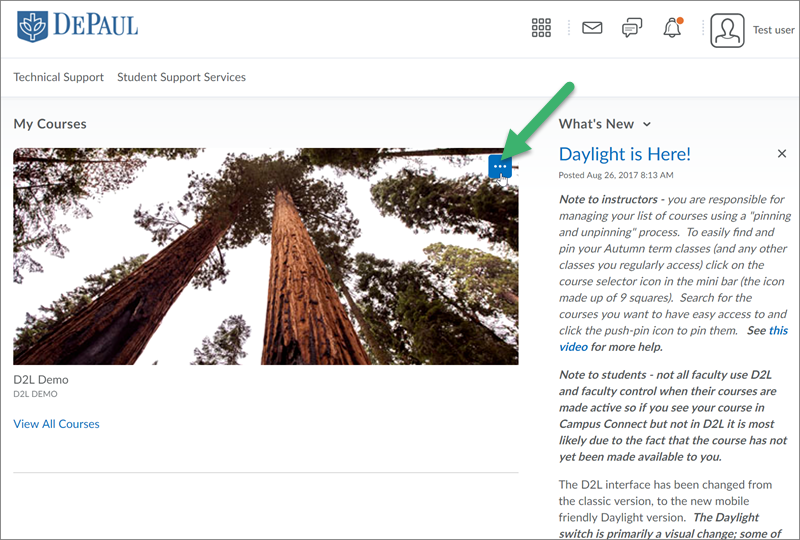**Title: Detailed Description of DePaul University Landing Page**

**Image Description:**

This image is a rectangular landscape format, approximately the size of a laptop screen, displaying a landing page from DePaul University, predominantly showcasing a clean, white background interspersed with various shades of light gray. 

**Upper Section:**

1. **Top Left Corner:** 
   - Features the DePaul University branding. 
   - The logo consists of a blue shield icon with a white symbol resembling an ankh at its center.
   - "DEPAUL" is written in uppercase letters, with the "D" and "P" being larger than the other letters.

2. **Top Right Corner:**
   - Displays a row of six icons:
     - A grid of nine gray squares.
     - An envelope icon.
     - A double quote box icon.
     - A bell icon with a red dot indicating unread messages.
     - A generic avatar icon depicting a head and shoulders silhouette.
     - The label "test user" in small font.

A thin light gray underline extends horizontally across the image demarcating the top navigation section from the content below.

**Main Content Area:**

1. **Left Panel:**
   - Contains two sections of gray text, "Technical Support" and "Student Support Services," each word capitalized.
   - Below this concise content, encased within a light gray background, is the heading "My Courses" in bold gray font.
   - Beneath the heading, there's a wide rectangular image, approximately two and a half times as wide as it is high. The photo captures towering trees from a ground-up perspective, revealing their trunks, leaves, and glimpses of the sky.

2. **Overlay Elements on Image:**
   - A blue square with three white horizontal dots located in the upper right corner of the tree image.
   - A medium green, thick arrow overlays the image, positioned at a 45-degree angle pointing toward the blue square.

3. **Below the Image:**
   - The text "D2L demo" appears twice, first in larger font and then in smaller, all-capital font.
   - The phrase "VIEW ALL COURSES" is shown in small blue font.

**Right Panel:**

1. **Content Adjacent to the Tree Image:**
   - The section is left-justified and spans about the rightmost third of the image.
   - A gray header reads "What's New" accompanied by a downward-facing arrowhead.
   - Below this header, the text "Daylight is here!" is printed in large blue font, the largest on the page aside from the DePaul branding.
   - A black 'X' icon sits to the far right, allowing users to dismiss the notification.

2. **Informational Article:**
   - The article contains three paragraphs:
     - **First Paragraph (10 lines):** 
       - Begins with "Note to instructors" in bold, followed by italicized text discussing the management of the course list.
     - **Second Paragraph (6 lines):**
       - Entirely italicized and in bold, starting with "Note to students" and discussing faculty usage of D2L.
     - **Third Paragraph (4 lines and cut-off):**
       - Switches back to non-italicized font, beginning with "The D2L interface has been changed from" and then getting cut off mid-sentence, hinting at a continuation.

This comprehensive layout offers a structural understanding of DePaul University's landing page, ensuring a specific and clear depiction of each visual and textual element.